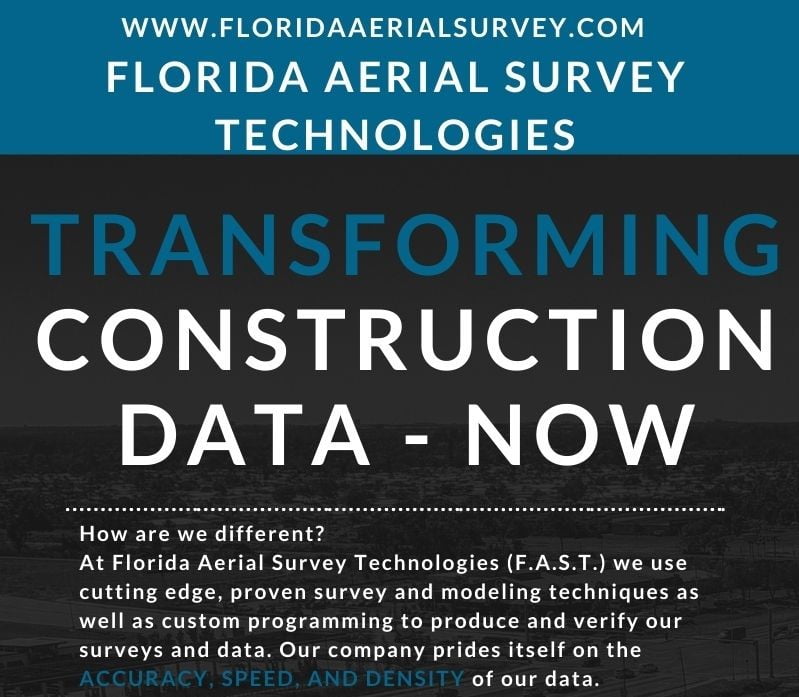The image is a digital flyer or poster with a professional layout, featuring prominent branding and detailed information about the services offered. At the very top, there is a blue banner with three lines of white text that read: "www.FloridaAerialSurvey.com," "Florida Aerial Survey Technologies." The rest of the image has a black background adorned with multiple lines of text. The top line is in blue, stating "Transforming," followed by two lines of white text: "Construction Data Now." Beneath these, a dotted white line separates the header from the smaller informational text below.

The finer white text reads: "How Are We Different? At Florida Aerial Survey Technologies, FAST, we use cutting-edge proven survey and modeling techniques as well as custom programming to produce and verify our surveys and data. Our company prides itself on the accuracy, speed, and density of our data," with the words "accuracy," "speed," and "density" emphasized in bold blue fonts. In the background, there is a subtle, blurred image depicting what appears to be a cityscape with roads and buildings, adding a contextual visual element to the flyer.